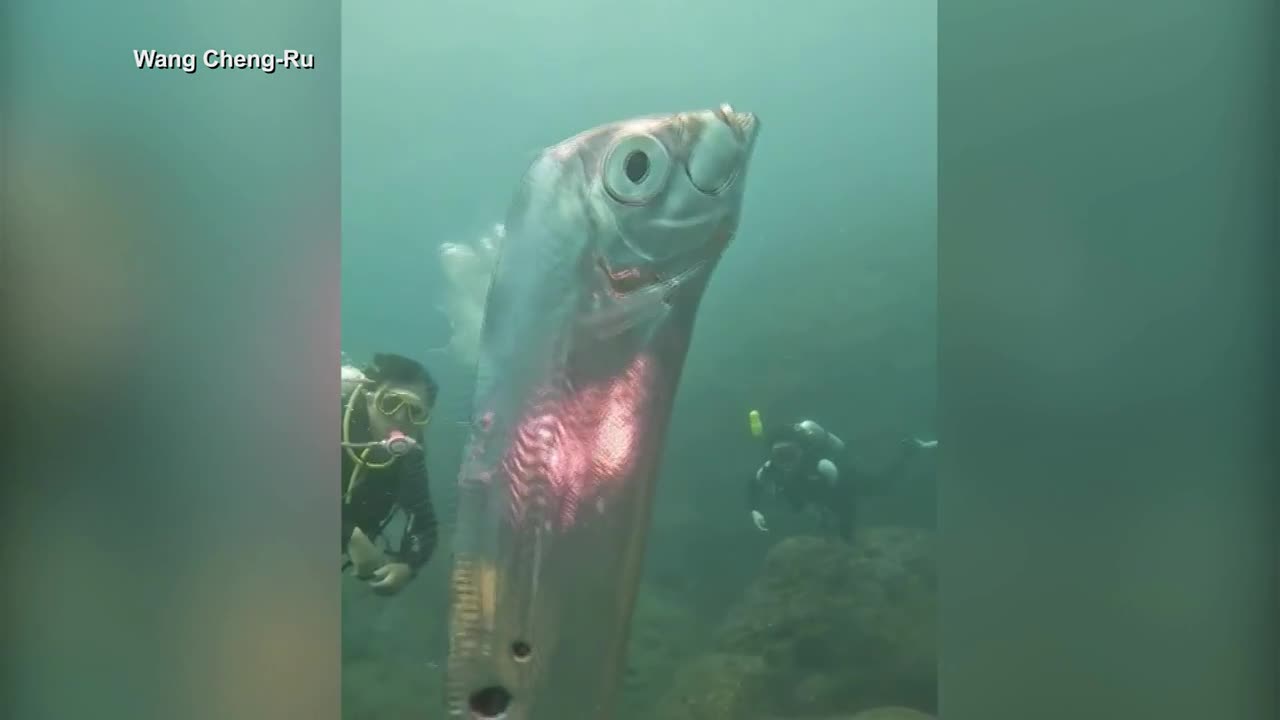The image portrays an underwater scene with a greenish cast, indicative of a deep ocean setting without sunlight. In the foreground, a large, uniquely shaped fish stands almost vertically with a metallic gray body accented by fluorescent pink and yellow hues, particularly noticeable along its spine and internal glow. This fish dominates the center of the image. To the left, a scuba diver equipped with a tank and full diving gear appears closer and seems to be observing the fish, while another diver in similar gear is slightly more distant to the right, seemingly swimming towards the fish. Both divers, submerged in the cloudy, blue-green water, explore an ocean floor scattered with dark rocks and formations. The left corner of the image is annotated with the text "Wang Chin Dash Roo," with some variations in spelling noted, against a bordered background with pink, peach, and gray colors. Blurred borders at the sides of the photo give it a soft frame, drawing focus to the central underwater tableau.